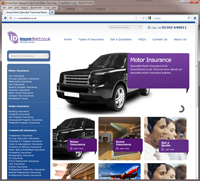Here is a detailed and cleaned-up caption based on the provided information:

"This image portrays a somewhat blurry screenshot of an application or website interface, predominantly themed in purple. The company logo, resembling a purple leaf and containing the initials 'ID,' is positioned at the top. Though the explanation of 'ID' is present just to the right of the logo, it is not readable. Below the logo, there are six navigational tabs available for exploration.

On the left side, there is a text box for user input followed by a lengthy blue column. This column appears to list numerous options arranged under three subheadings, all of which are unfortunately unreadable. Each subheading contains multiple items beneath it.

The right side of the interface prominently features a large black SUV set against a white background, with a purple quote box labeled 'motor insurance'. Below this, three additional lines of text are present but not decipherable. Underneath the section displaying the car, there are three images. The first is a repeated image of the black SUV. The second image’s content is unclear. The third depicts three individuals, possibly telephone operators, engaged in phone conversations."